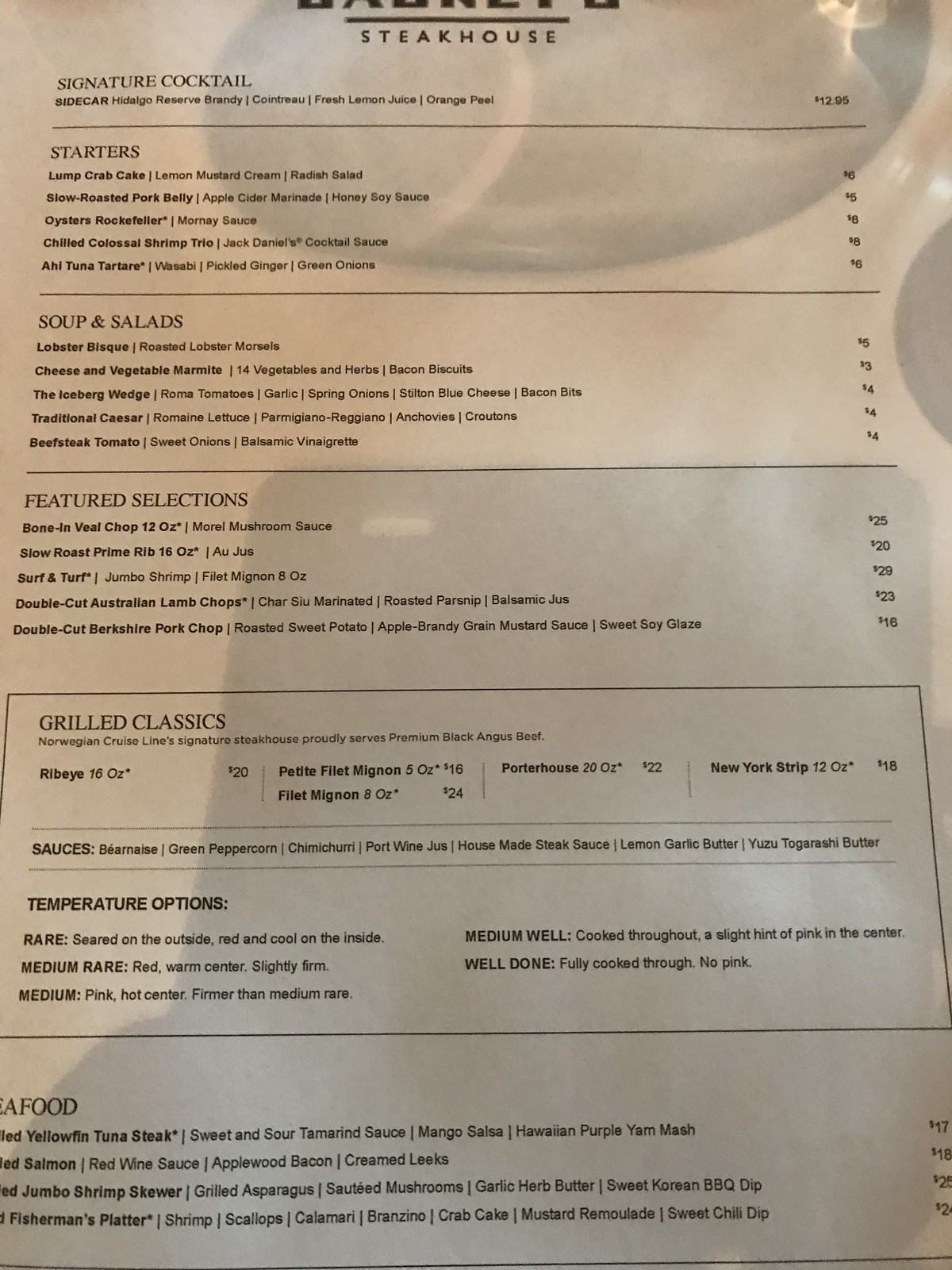This is a detailed caption for the image:

"The image features a page from a restaurant menu, printed on a sheet of white paper with black typed text. The menu is organized into several categories separated by straight black lines. Starting from the top, the legible categories include 'Soups and Salads,' 'Featured Selections,' and 'Grilled Classics,' followed by temperature options listed below the grilled classics section. The final category, 'Seafood,' is partially cut off in the image. Each item under these categories is listed with prices aligned to the right margin, though the prices are too small to be read clearly. Under 'Soups and Salads,' the offerings include Lobster Bisque, Cheese and Vegetable (illegible), Iceberg Wedge, Traditional Caesar, and Beefsteak Tomato. The 'Featured Selections' category lists Veal Chop, Prime Rib, Surf and Turf, Australian Lamb Chops, and Double Cut Pork Chops. The 'Grilled Classics' features Ribeye, Filet Mignon, Porterhouse, and New York Strip, with temperature options ranging from Medium to Well Done."